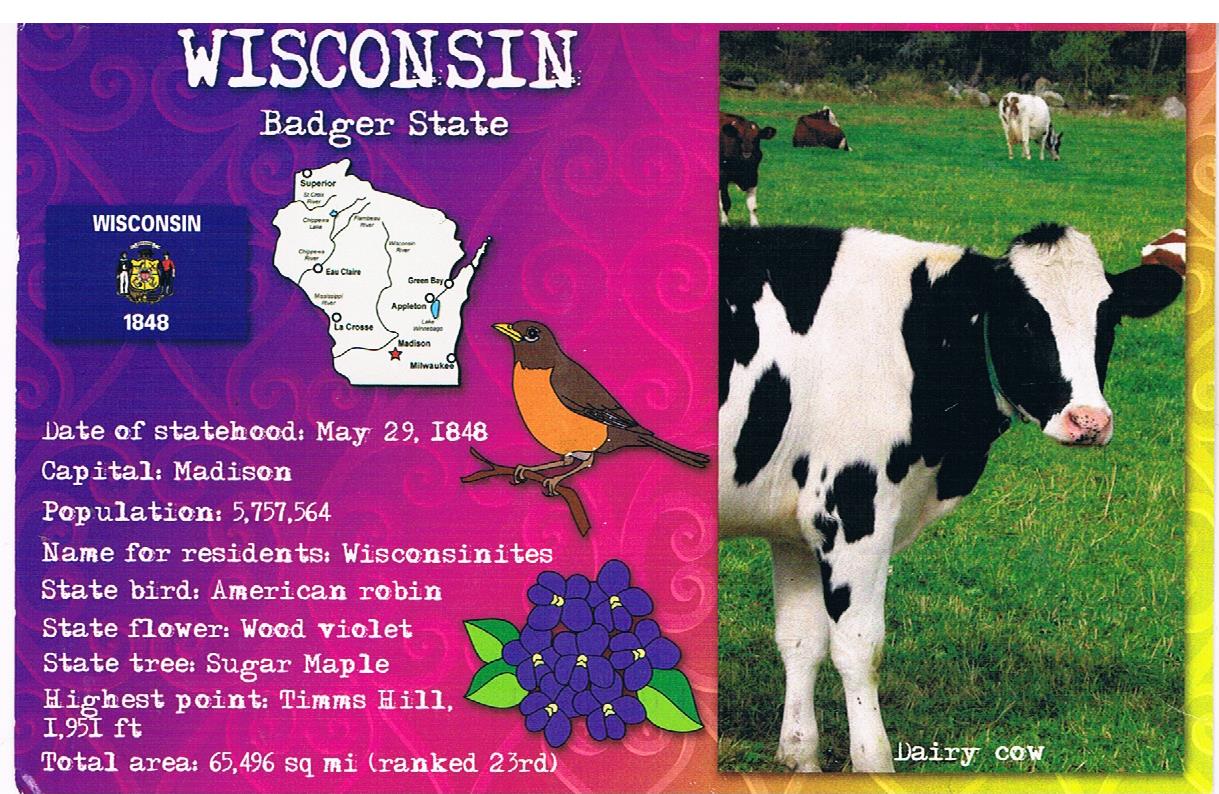The image is a vibrant and detailed infographic that appears to be a postcard advertising Wisconsin. It has a colorful background with a gradient of purple, pink, yellow, and hints of orange. On the left side is a purple graphic design resembling a decorative fence with heart patterns, set against various shades of purple. Prominently displayed in large, spray-paint style white text are the words "Wisconsin" and "Badger State."

Embedded within the left section, the infographic features a white, 2D map of Wisconsin showing various city names and black lines, though the text is mostly unreadable, with "Green Bay" faintly discernible. To the left of this is the Wisconsin state flag, depicting a blue field with "Wisconsin" and "1848" in white text, and a central yellow emblem flanked by two figures.

Additional Wisconsin facts are listed in smaller, spray-paint style text: "Date of Statehood: May 29, 1848," "Capital: Madison," "Population: 5,757,564," "Name of Residents: Wisconsinite," "State Bird: American Robin," "State Flower: Wood Violet," "State Tree: Sugar Maple," "Highest Point: Tim's Hill, 1,951 feet," and "Total Area: 65,496 square miles, Ranked 23rd."

Illustrations include a cartoonish depiction of an American Robin with a brown body, yellow beak, and orange chest perched on a brown branch, and a bouquet of Wood Violets, displaying several purple flowers with accompanying green leaves.

On the right side of the infographic is a high-quality photograph of a black and white dairy cow positioned toward the center, with the head to the right. Below this image, the text "Dairy Cow" is displayed. The background shows a green field with four other cows—black and white plus a couple of brown cows—lazing and grazing.

Overall, the infographic blends informative text with colorful, illustrative elements to portray key details and symbols of Wisconsin.